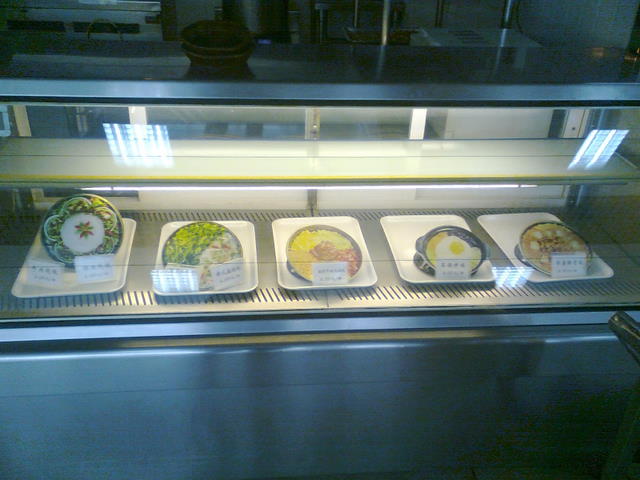The image captures an indoor display within what appears to be a restaurant or possibly a grocery store with a cafeteria-like setting. The primary focus is a long, stainless-steel cooler or food display unit with glass panels covering and protecting the food. Inside, there are five distinct dishes artfully arranged on plastic trays and presented in bowls or on plates. The display has a light blue tint, with focused lighting illuminating the vibrant food items.

From left to right, the dishes include a green and white salad that is propped up, another green and white dish, a yellow and red starchy item that appears to resemble potatoes, a dish featuring a sunny-side-up egg on a yellow-golden base, and a brown and white dish. The food labels, written in Asian script, are placed on the plexiglass, indicating each dish's name or contents. 

The cooler sits in a darker environment with reflective lights adding a subdued glow, while the background shows hints of kitchen tools and appliances, giving a sense of a working kitchen space. This detailed presentation suggests that these could be dishes available for purchase, perhaps intended for lunch or takeaway.